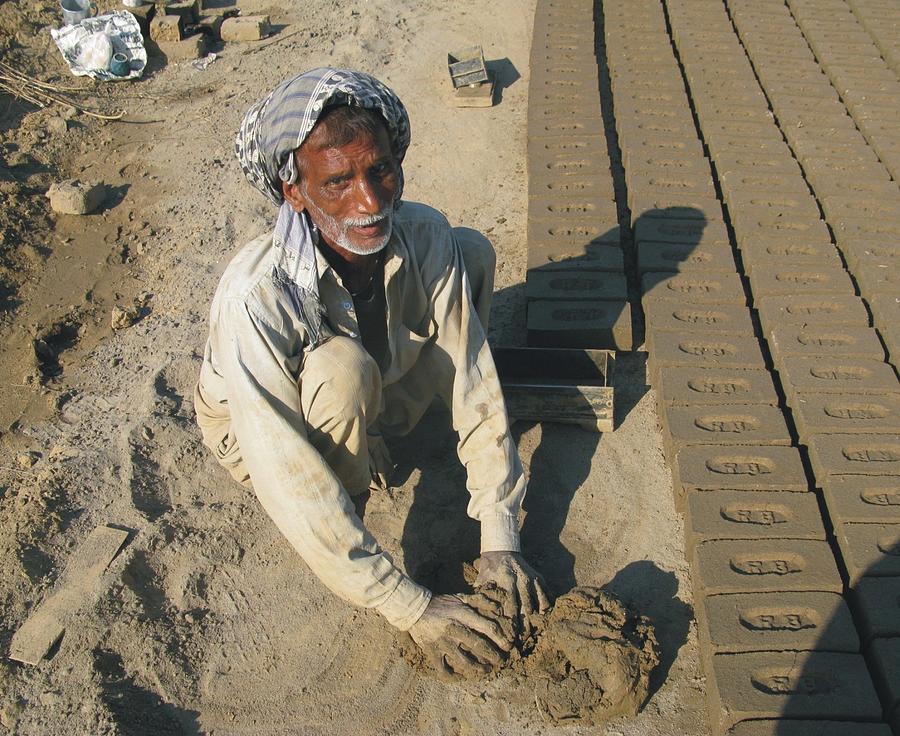In this image, a tan-skinned man of Indian or Middle Eastern descent is seen kneeling on the left side, meticulously crafting bricks on a sandy ground. He has a distinctive appearance with dark hair, a white beard, and a white goatee. His attire includes an all-white long sleeve shirt that's unbuttoned, revealing his chest, and tan or khaki-colored pants. His head is wrapped in a white and blue striped turban, adding to his unique look. His clothing and hands are quite dirty from handling the sand and clay.

In front of him, he is diligently molding bricks from dark tan sand mixed with clay. His hands are extremely dirty, coated in the dry, light brown clay, making them appear almost white. The bricks he is making are embossed with "RB" in an oblong shape. Surrounding him are various brick-making tools, including a wooden box mold and a silver pail. Piles of sand, rocks, and dirt are visible behind him, alongside neatly aligned rows of dark tan bricks that stretch vertically into the distance, all uniformly stamped with "RB." The scene intricately captures the man's dedication to his craft in this traditional brick-making environment.